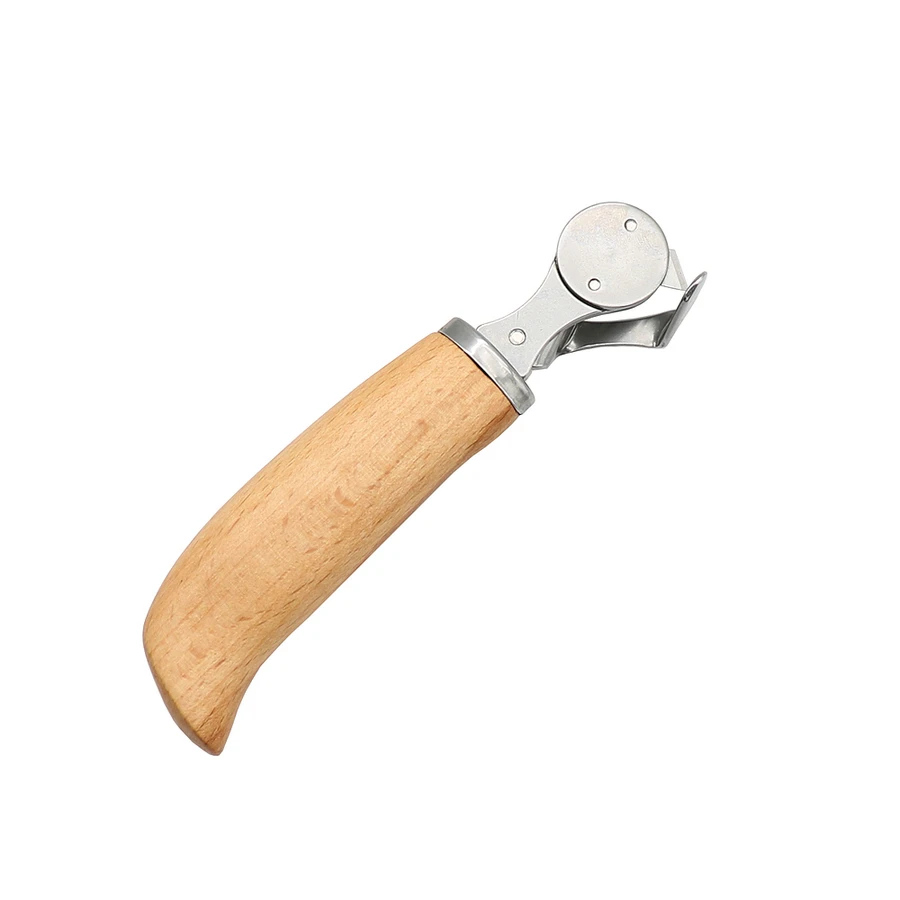This detailed close-up image showcases a vintage hand-operated can opener. The tool prominently features a light wooden handle designed for a single-hand grip. Affixed to the top of the handle is a silver metallic component. From this metal fixture, a rectangular section extends upwards, transitioning into a circular area. Emanating from this circle is a small triangular blade. Beneath the blade, another metallic part protrudes upwards, seemingly intended to interact with the blade for the can-opening function. The entire apparatus, set against a stark white background, lacks visible mechanisms such as a turn knob, which leaves some ambiguity regarding its exact usage method. Despite the uncertainty around the specific operation, the intricate design and materials suggest it is an old-fashioned can opener.